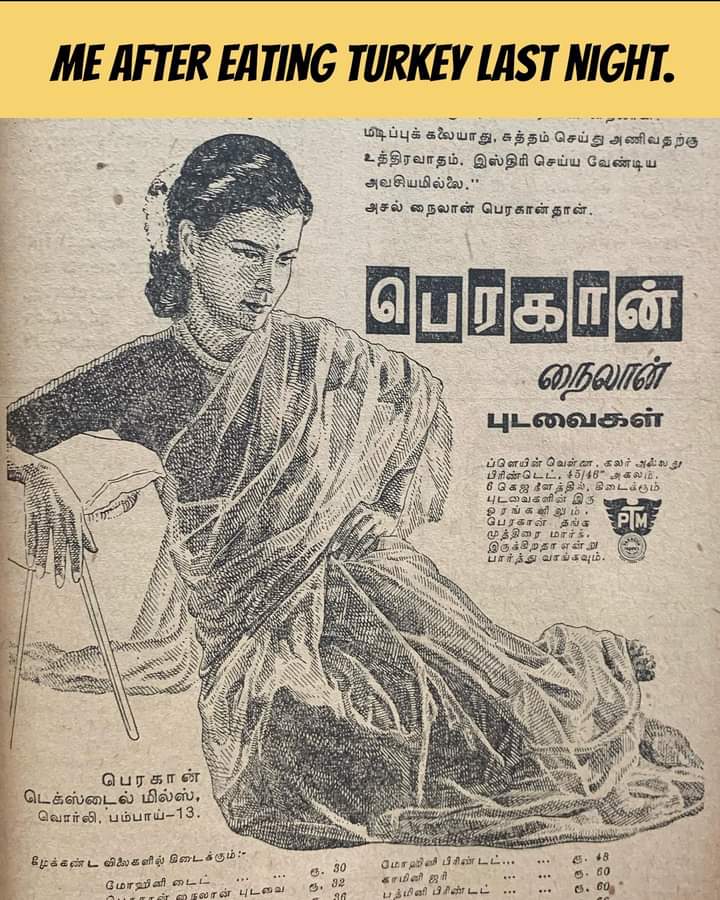The image is a digitally enhanced, black-and-white photograph set against what appears to be an old South Asian newspaper ad, with text in an unfamiliar language surrounding the central image. The focal point is an artistic photograph of a young woman dressed beautifully in traditional attire, her hair neatly styled. She sits in a languid pose on the floor, her head tilted downwards, eyes half-closed as if exhausted, with one arm resting on a stool beside her. Over the top of the image, a bright orangey-yellow banner with black, bold, all-capital letters humorously reads, "ME AFTER EATING TURKEY LAST NIGHT," suggesting a state of post-meal lethargy. The overall effect blends a contemporary meme's humor with vintage aesthetics, creating a whimsical commentary on the aftermath of overeating.